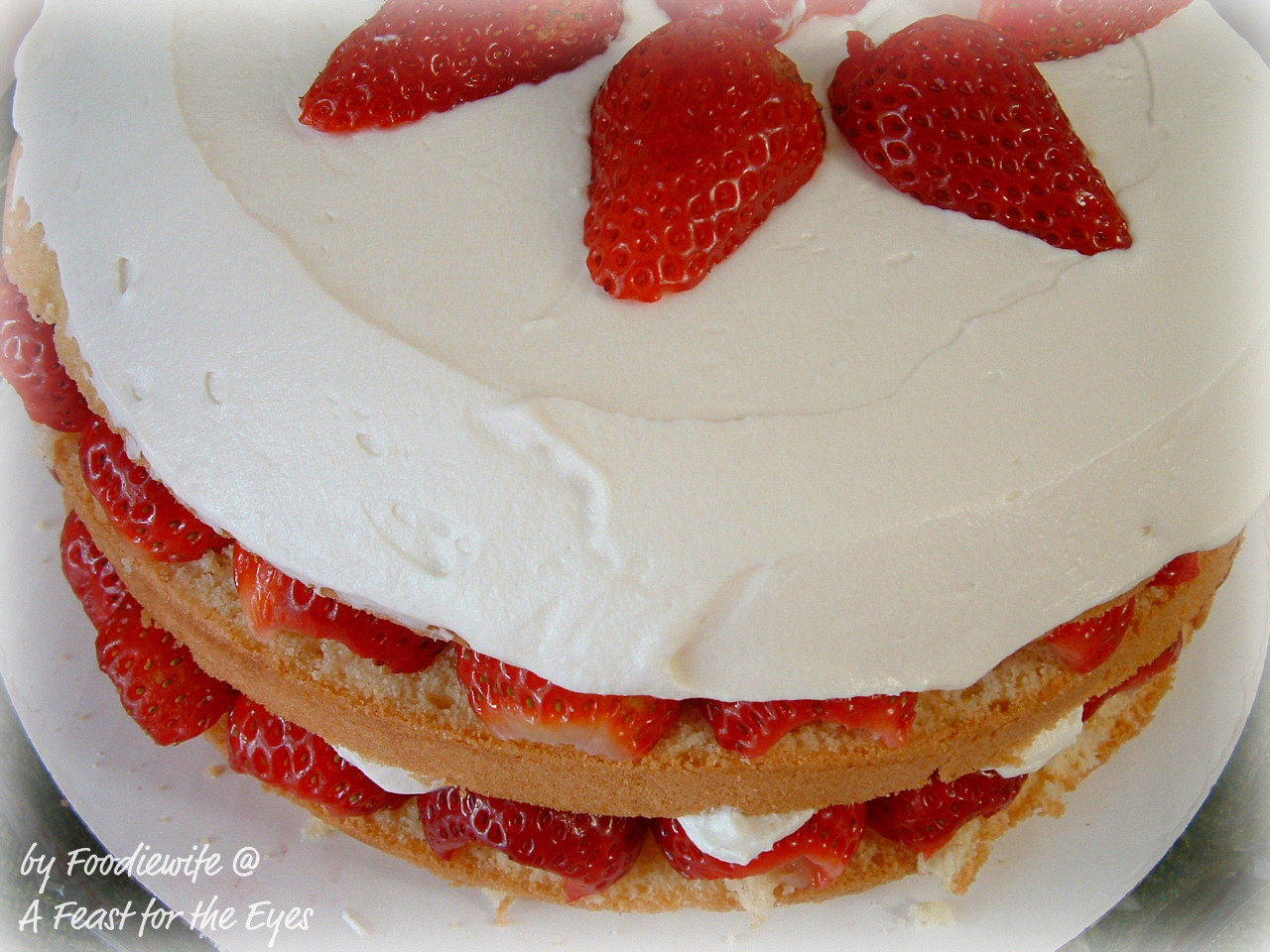This mouthwatering, homemade strawberry shortcake features two to three layers of light tan cake, generously layered with dense and juicy red strawberries and velvety whipped cream. Each tier alternates between the cake and a rich mixture of strawberries and whipped cream that oozes out from the sides. The top layer is adorned with a creamy dollop of whipped cream and a handful of whole strawberries, creating a feast for the eyes. Presented on a white plate, this delicious dessert is illuminated by a bright white light from the left, highlighting its delightful textures and colors against a grayish background. The cake, shared by "foodie wife at feast for the eyes," exudes homemade charm and culinary expertise, making it an irresistible treat reminiscent of classic strawberry shortcake.